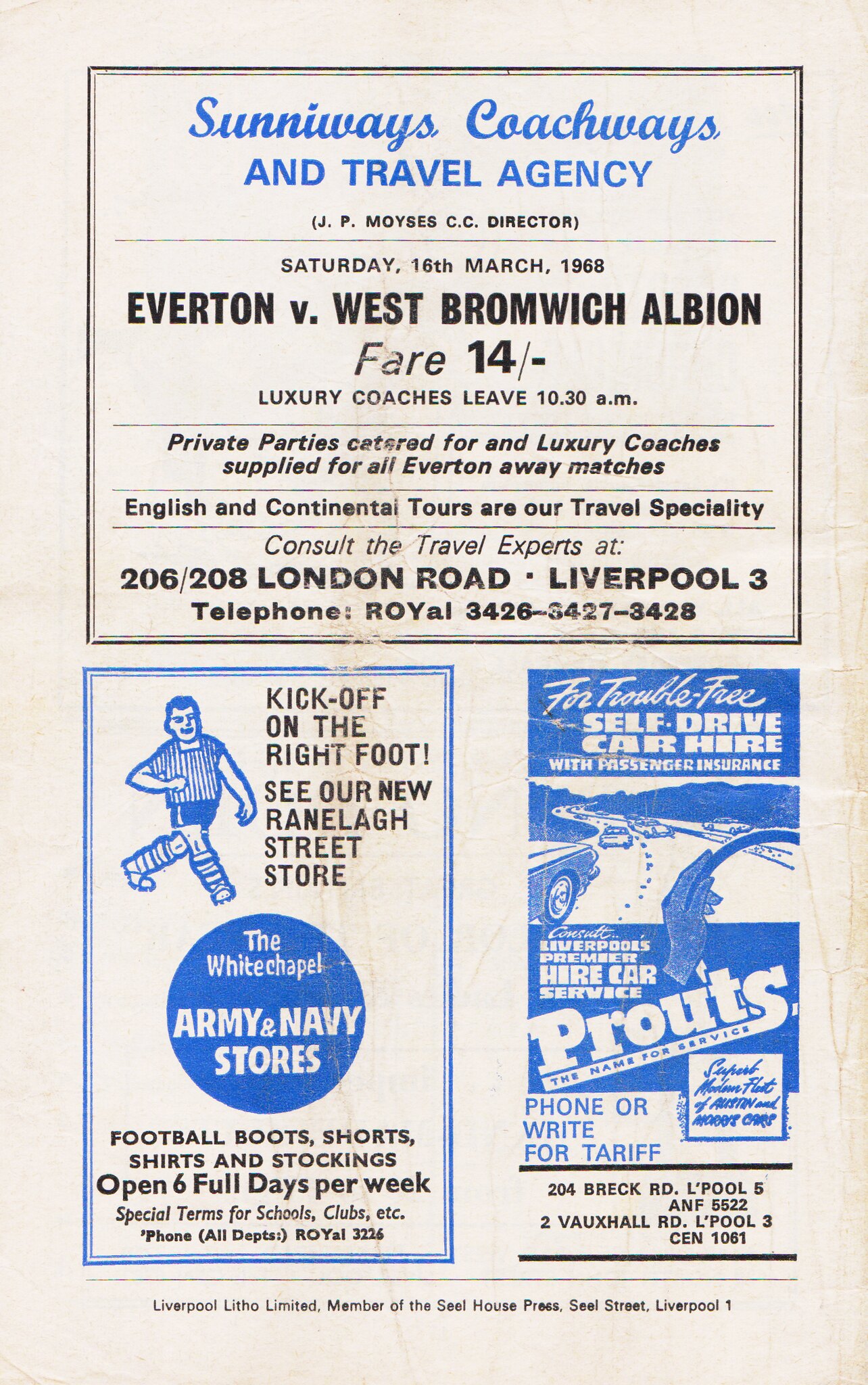The image depicts a vintage printed flyer, slightly weathered, against an off-white background featuring black and light blue ink. Dominating the top section is an advertisement for Sunnyways Coachways and Travel Agencies, with the director's name mentioned below. It prominently displays the date, Saturday, 16 March 1968, and advertises a football match between Everton and West Bromwich Albion. The flyer details the availability of Fair 14 luxury coaches departing at 10:30 a.m. Additionally, it offers services for private parties and emphasizes their expertise in arranging English and continental tours. Their contact details are listed as 206-208 London Road, Liverpool 3, with the telephone numbers Royal 3 4263, 4273, and 4283. The lower part of the flyer contains two predominantly blue advertisements: one for Army and Navy stores located in Whitechapel, England, and another for Prouts, a car rental service in Liverpool. The imagery and fonts evoke a sense of nostalgia reminiscent of old printed materials from the mid-20th century.